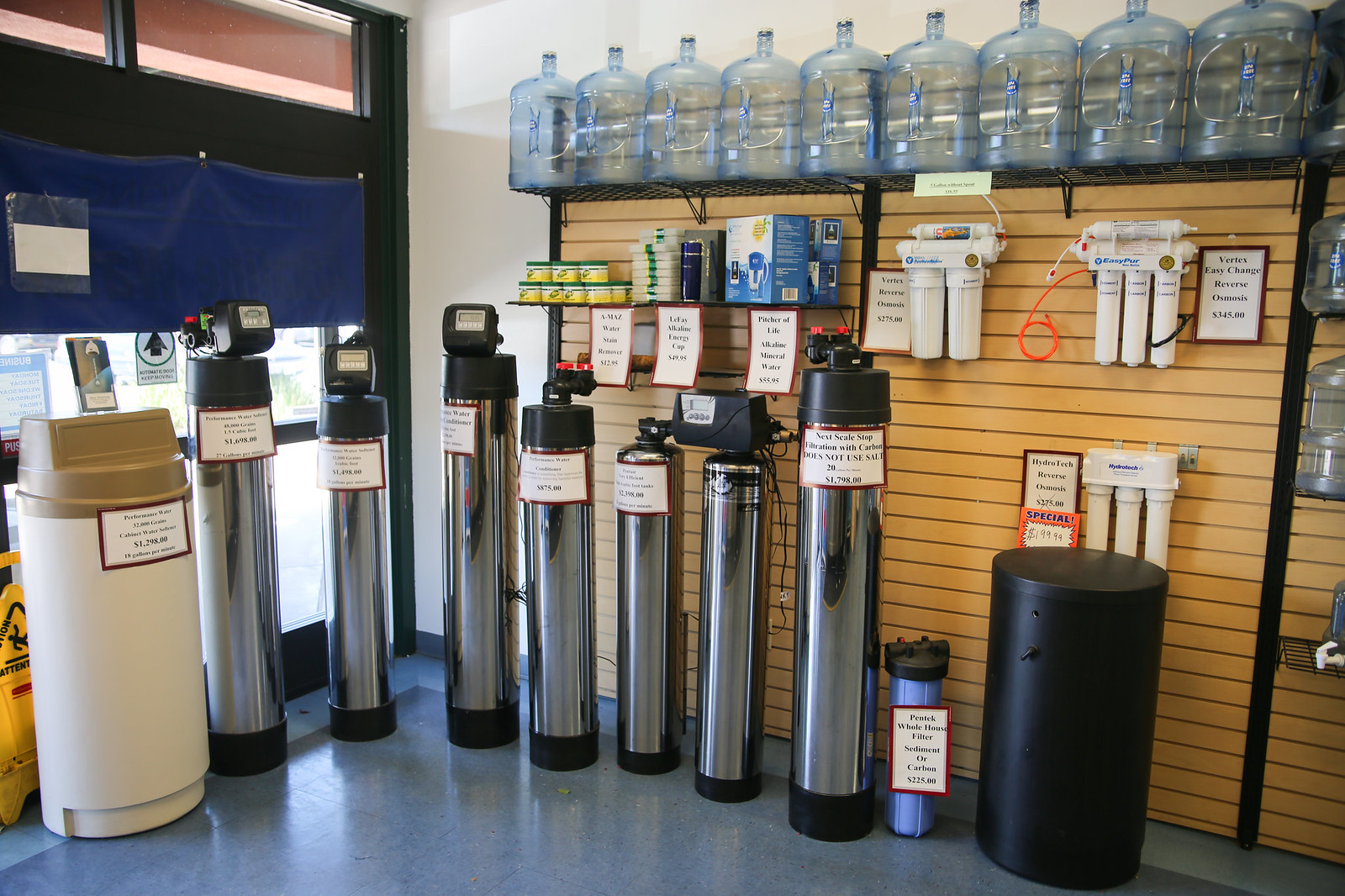This color photograph showcases an indoor scene, likely a section of a store or a factory specializing in water filtration systems. Prominent in the image are several tall, silver cylindrical water filters standing on a bluish-grey marble floor. These cylinders, potentially stainless steel, feature black tops and bottoms, and each has a white sign with a red border, offering details about their specifications and prices. The closest sign is partially readable, advertising a filtration system for $1,798, with additional text promoting its features.

Adjacent to these silver filters on the left, a cream-colored cylindrical object with a brown top, possibly a trash can, is also labeled with a similar sign. A large black cylinder, shorter and wider than the others, appears further to the right, accompanied by a tiny blue cylinder. 

The background reveals a brown slatted wooden wall used as a display area for smaller water filters, typically arranged in sets of two or three. These smaller filters are predominantly white and have signs beside them. Additional items, such as a blue box on a shelf, a set of yellow and green boxes, and smaller yellow and green boxes, are also visible. Above these displays, a row of tall, translucent five-gallon water jugs with narrow necks and taps aligned horizontally stands out.

To the left side of the scene, a window or possibly a framed opening is partially covered by a dark blue shutter pulled halfway down. The top part of the roof is painted red with two white lines running through it, and the wall above the display area seems to be a lighter grey compared to the floor.